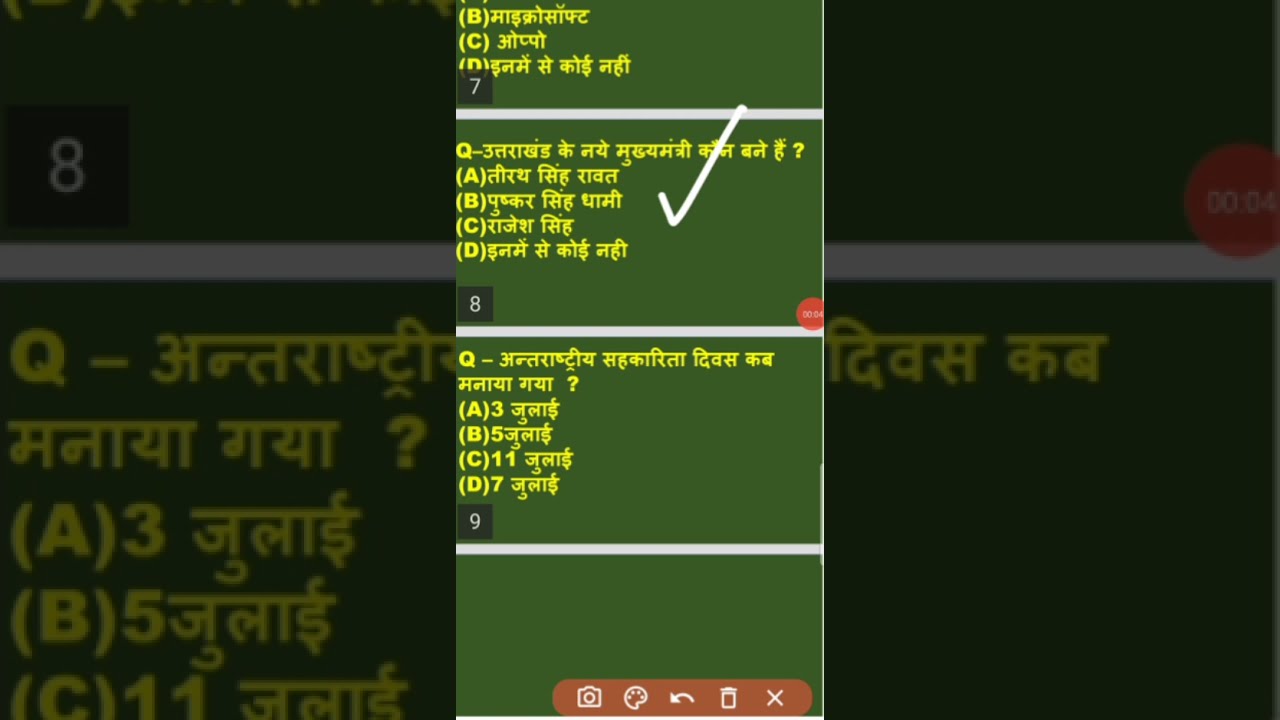The image appears to be a screenshot from a smartphone, displaying what seems to be a test or quiz with multiple-choice questions. It is divided into four vertical columns, each separated by a thin white line and set against a green background reminiscent of a green chalkboard texture. The top three boxes, marked with the numbers 7, 8, and 9 in their bottom left corners, are visible, while the fourth is cut off. Each question is accompanied by multiple-choice answers labeled with the letters A, B, C, and D, written in yellow text. The second box down features a hand-drawn white checkmark, suggesting an answer has been marked or graded, likely using a stylus. The language of the text appears to be Middle Eastern, possibly Arabic or Hindi, but the specific dialect remains unclear. Additionally, there is a small red recording button on the right-hand side and a brown toolbar at the bottom with various icons, including a camera, paintbrush, undo, trash can, and close (X) icons. The image is framed within a darkened and enlarged version of itself, which further emphasizes the main content in the center.